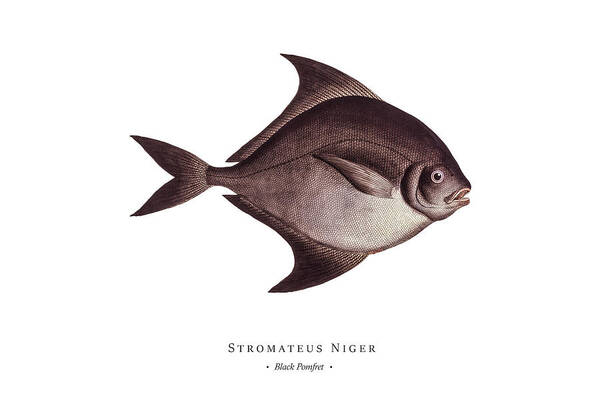This detailed drawing on a rectangular white background showcases a fish identified as Stromatus Niger, or Black Pomfret, as noted by the black text at the very bottom center, framed by asterisks. The fish is depicted facing right and measuring roughly two inches in length. Its disc-shaped body features a large ridge on both its back and stomach, with two prominent, spiked dorsal fins and a symmetrical ventral fin creating a balanced silhouette. The fish's coloration transitions from a dark, almost black back to a silvery underside, while the fins display a gradient from white at the bottom to black at the top. A thin black line runs the length of its body, from the base of its almond-shaped tail fin to its head. The tail fin forms a distinct V shape at the end of its streamlined form. Notable details include a gill situated near the large, rounded eye and a small, open mouth positioned at the narrowest point of its head.